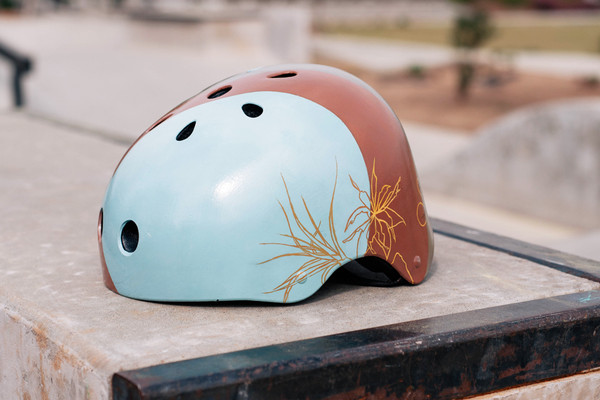This color photograph captures a close-up of a helmet, likely used for skating or biking, resting on a concrete bench lined with metal that is scratched and rusted. The helmet features a light blue back and a red front, adorned with yellow floral and leaf patterns. It is perforated with numerous ventilation holes. The background is heavily blurred, suggesting the setting is an outdoor skate park, with visible concrete ramps and possible hints of dirt, plants, and indistinct figures, possibly people in motion. The concrete bench is dirty, adding to the gritty urban atmosphere of the scene.